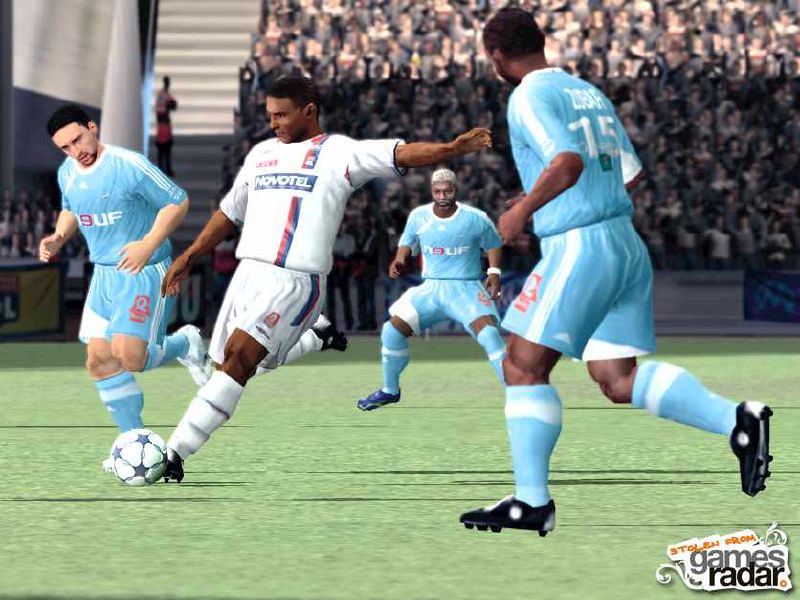The image depicts a video game screen showcasing an intense moment from a soccer match. A player dressed in a white uniform with red and blue stripes is about to kick a white ball adorned with blue stars, his leg poised in mid-air. He wears a blue banner across his chest that reads "NoVotel." Surrounding him are three opponents clad in light blue uniforms with white accents and vertical lines. Their jerseys are emblazoned with "N9UF," with the '9' in red and the other letters in white. In the bottom right corner, an icon indicates the image is "Stolen From Games Radar," and a white tag overlays the bottom of the screen.